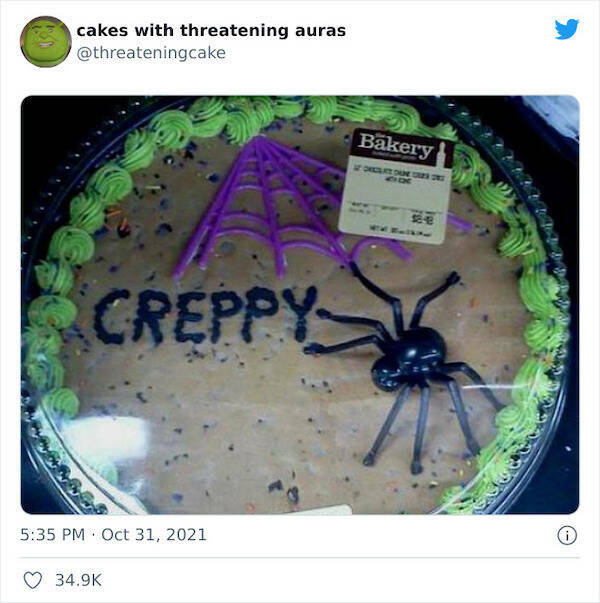This screenshot captures a social media post with a visibly unsettling cake in the spotlight. The overall background is white, emphasizing the central image – a cake designed to resemble the character Shrek. At the upper left corner, the text "Cakes with Threatening Auras" is displayed, framing the peculiarly eerie scene. The upper right corner features the Twitter icon and the handle @threateningcake, suggesting a profile dedicated to sharing intimidatingly bizarre cake designs.

The cake in question appears to be fashioned with green icing and adorned with chocolate chip cookie features. Its aura of creepiness is amplified by a plastic spider on the right side and decorative purple spider webs at the top. To add to its quirky charm, the word "CREPPY" is inscribed on the left side in place of "creepy." A price tag labeled "bakery" indicates that it costs around $8.48, although the full description is partially obscured.

In the bottom left corner, the post's timestamp reads 5:35 p.m. on October 31st, 2021 – fittingly, Halloween. This peculiar cake has garnered significant attention, amassing 34.9 thousand likes, likely because of its odd misspelling and overall eerie presentation.